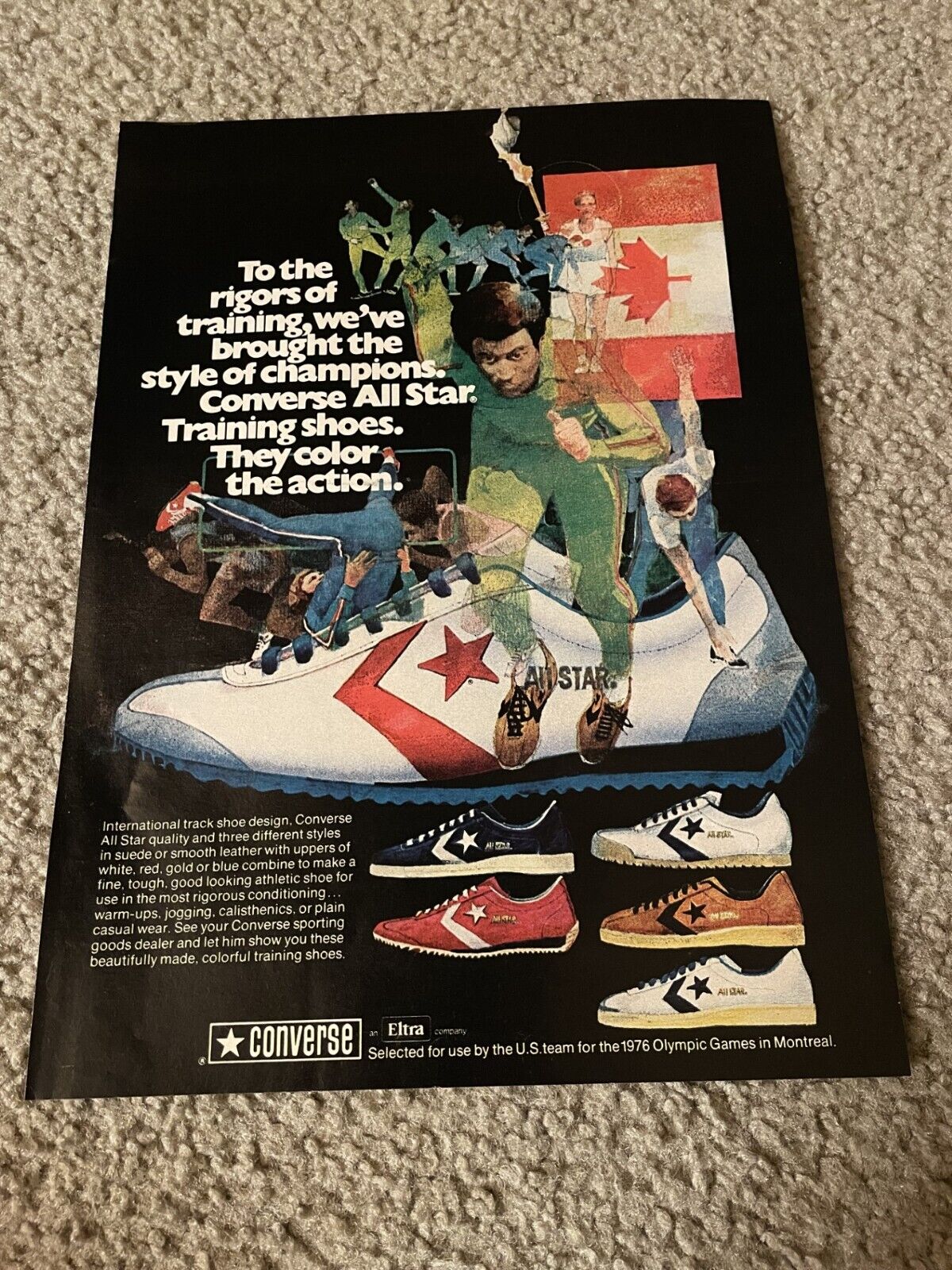This photograph showcases a vintage poster from the 1976 Olympics, placed on a tan shag carpet, possibly within a home. The poster, primarily black, prominently features a large image of a white Converse All-Star training shoe with blue laces and a red star emblem at its center. Surrounding the shoe are images of various Olympic athletes participating in different sports, with a Canadian flag—a white flag with red borders and a central red maple leaf—situated in the upper right corner.

Above the athletes and the shoe, white text reads: "To the rigors of training, we've brought the style of champions. Converse All-Star training shoes. They color the action." Toward the bottom of the poster, a series of additional Converse shoes in diverse colors—red, white, black, brown, and half-white—are displayed. A detailed caption to the left highlights the attributes of the shoes, stating: "International track shoe design, Converse All-Star quality, and three different styles in suede or smooth leather with uppers in white, red, gold, or blue combination to create a fine, tough, good-looking athletic shoe for use in rigorous conditions—conditioning, warm-ups, jogging, calisthenics, or casual wear. See your Converse sporting goods dealer and let him show you these beautifully made color training shoes."

At the bottom center of the poster, the Converse logo appears, enclosed within a white rectangular box, accompanied by the text indicating that these shoes were selected for use by the U.S. team at the 1976 Olympic Games in Montreal.